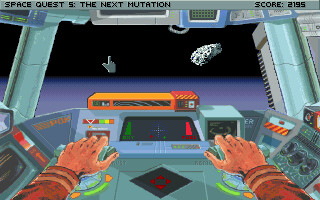This image appears to be a detailed screenshot from an old, cartoony video game, likely from 20 to 30 years ago, called "Space Quest 5: The Next Mutation," as indicated by the text at the top of the screen along with a score of 2195. The setting is the interior of a spaceship cockpit, depicted with less realism and more caricatured style characteristic of older games. The cockpit showcases various screens, switches, and buttons. The perspective is from the pilot's viewpoint, showing two hands clad in red long-sleeved shirts with yellow stripes, manipulating a joystick. Outside the large cockpit window, the blackness of outer space is visible, dotted with spacecraft, a meteor towards the right, and a blue expanse that could be Earth or another planet's atmosphere. Additionally, a hand making a backwards L shape with its fingers appears floating in space, adding to the whimsical, illustrative nature of the game's visual design.